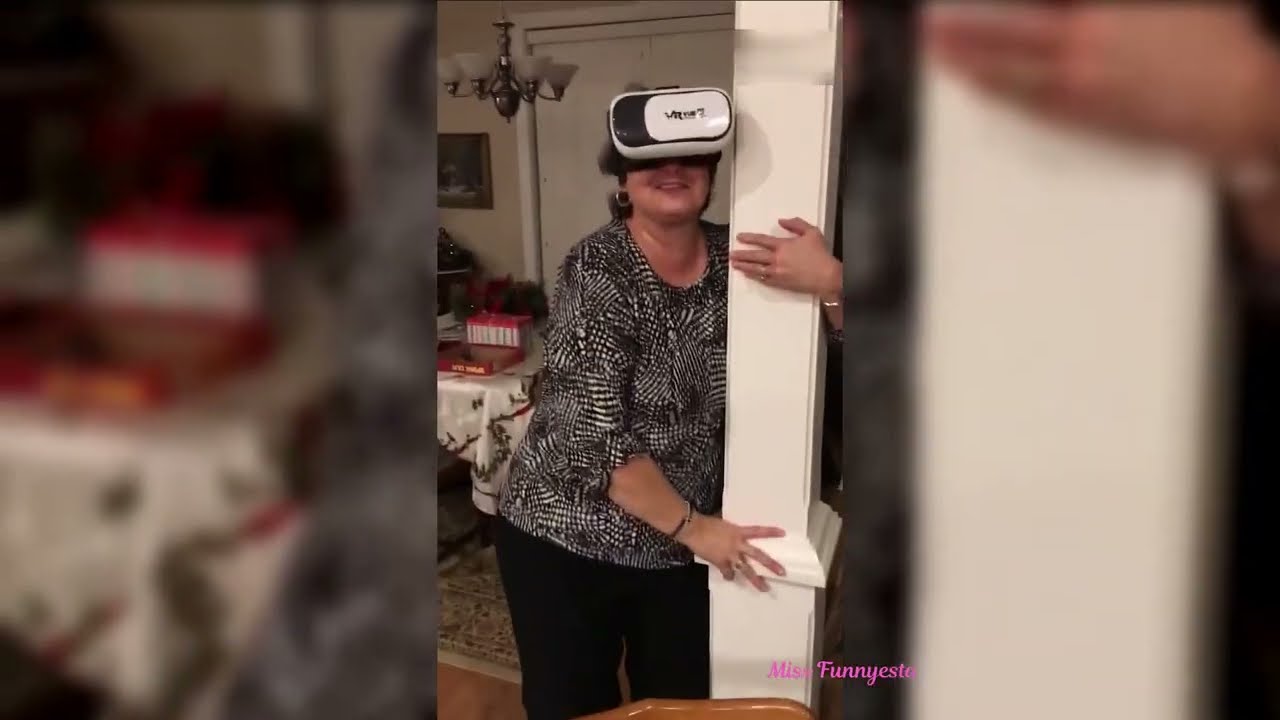In this image, a middle-aged Caucasian woman, possibly in her 50s or 60s, is experiencing a virtual reality game for the first time. She is at the center of the horizontal, rectangular photo, with the left and right sides blurred to emphasize her presence. The woman is slightly heavy-set and wears a black blouse with some white detailing, paired with black pants. She holds a white column, likely for balance, with both arms wrapped around it, and a virtual reality headset obscures her eyes. She has a tentative smile on her face, reflecting a mix of curiosity and amusement.

The setting appears to be a domestic interior, specifically a room decorated for Christmas. Behind the woman, there is a table covered with a white tablecloth featuring a green and red design, possibly indicating a holiday theme. On the table are some boxes and a present. A chandelier-style light fixture with four bulbs hangs above the table, and the light-colored wooden floor beneath is partially covered by a fringed rug. The wall in the background is white, adorned with framed pictures, and there is a door visible to the right.

Additionally, the photo features an artistic touch where the original image has been enlarged and darkened to create a blurred background visible on both the left and right sides. In the bottom-right corner of the image, there is text in pink lettering reading "Ms. Fuddyista" or “Miss Funny something,” suggesting a playful title for the scene.